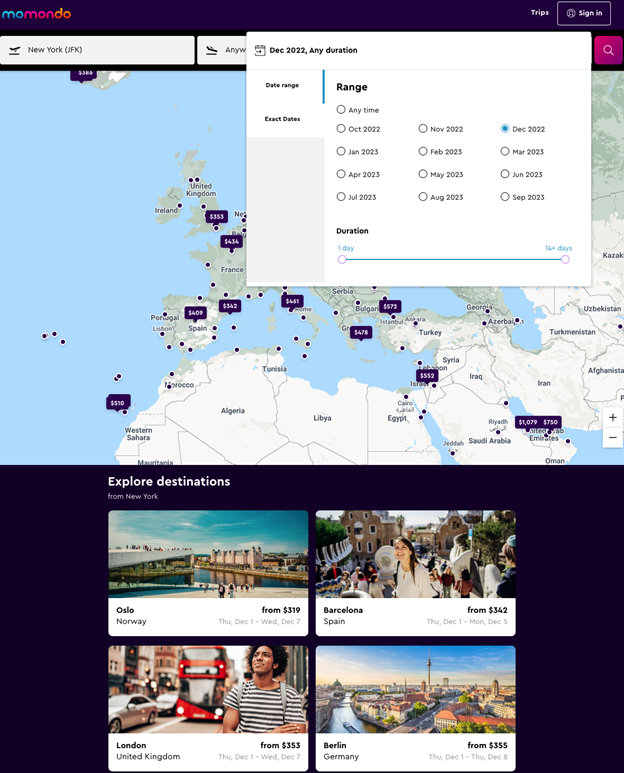In the upper left corner of the image, there is a logo that reads "Mo Mondo." The letters "M" and "O" are in light blue, while the letters "M," "O," and "N" are in dark pink. The letters "D" and "O" feature an ombre effect transitioning from dark pink to light orange. Below the logo, there is a search field with the text "NEW YORK (JFK)" in all caps. To the left of this search field is a gray airplane icon. To the right of the search field, partially obscured by an overlay, is the text "NEW," likely part of the word "ANYWHERE."

The overlay is a long white rectangle with a light gray header at the top. Within the header, there is a calendar icon on the left and bold black text that reads "DEC 2022, any duration." Directly beneath the header, a menu is positioned on the left side of the overlay. The first two menu options, titled "Date ranges" and "Exact dates," are displayed against a white background and a blue scrollbar is visible to the right, which may indicate a selected option.

To the right of the menu options is the word "range" in bold black lettering, under which are tick boxes labeled with various time frames: "Any time," "OCT 2022," "January 2023," "April 2023," "July 2023," continuing up to "September 2023." At the bottom of the overlay, the word "duration" appears in bold black text, accompanied by a scroll bar where a small white icon can be adjusted to set the desired trip length.

In the background of the image, a map is visible. The map predominantly features light blue areas representing water and beige with green areas denoting land. At the bottom of the map, the country names "Algeria" and "Libya" are marked in black lettering, with Algeria appearing on the left and Libya on the right.